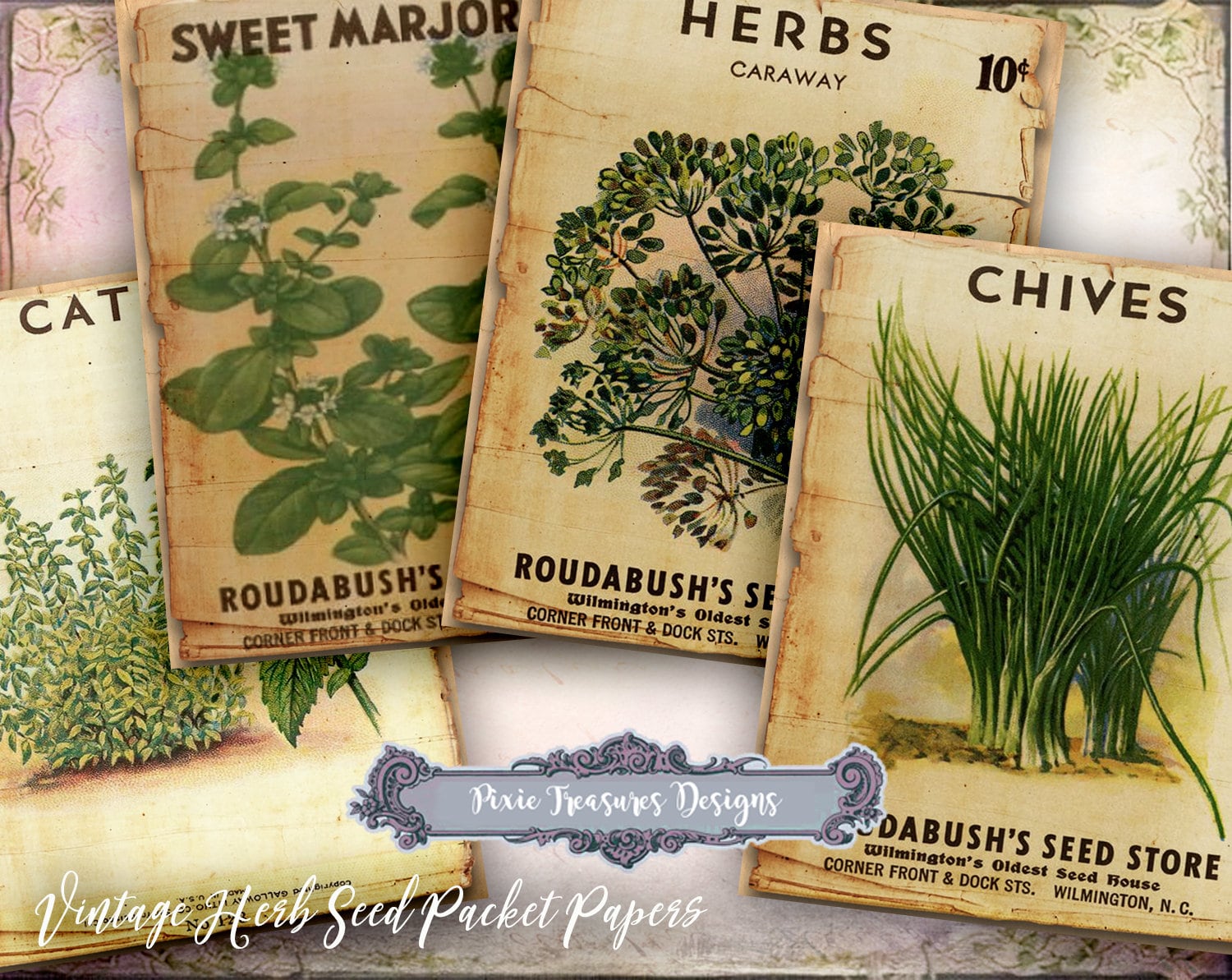This vintage-style illustration showcases a collection of four herb seed packets, meticulously arranged and overlapping on a parchment-like background adorned with leafy decorations. The packets, which are reminiscent of early 1900s publications, are fanned out, creating a layered effect that partially obscures some details. From right to left, the featured packets include Chives, characterized by tall, grass-like blades; Caraway, notable for its tiny protruding stems and priced at ten cents; Sweet Marjoram, displaying green tapered leaves and delicate white flowers; and Catmint (or Catnip), identifiable by the word "Cat" at the top. Each packet prominently displays the label "Roudabush's Seed Store," accentuated with the phrase "Wilmington's Oldest Seed House," and provides the location as "Corner Front and Dock Streets, Wilmington, North Carolina." The overall layout is framed by a circular banner at the center bottom that reads "Pixie Treasures Designs," and the bottom left corner is graced with the cursive inscription "Vintage Herb Seed Packet Papers," both set against a gray background with elaborate curlicues.